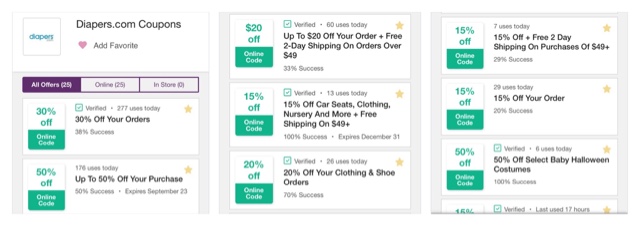The image displays the homepage of a website titled "Diapers.com Coupons." The top left corner features the diapers.com logo in blue. The main screen is populated with a series of white tiles, each highlighting various discount offers with green markers on the left-hand side, indicating the percentage off. For instance, one tile offers a 30% discount for an online code, allowing customers to save 30% on their order by using a specified voucher. 

The webpage is configured to display all 25 available offers, which customers can filter by online offers, in-store offers, or all offers. Currently, the display shows a range of discounts from 15% to 50% off. Specific offers include 15% off on car seats, clothing, nursery items, and mowers, 20% off with free 2-day shipping on orders over $49, and 20% off on clothing and shoe orders. 

The website not only provides discounts on diapers but also offers vouchers for a variety of baby products, making it a general-purpose online resource for baby-related discounts.